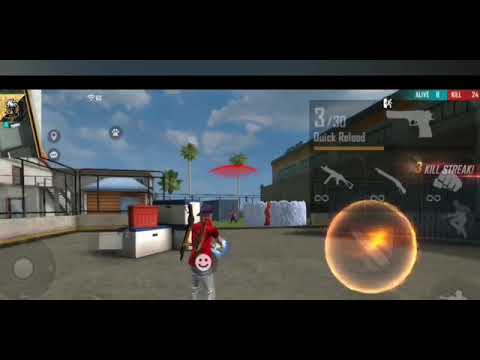The image is a detailed screenshot from a video game, likely taken on a computer or console. The primary focus is a central character standing on concrete, donned in a red shirt, gray pants with a smiley face on the back, and a gray hat. He carries a weapon that might be a crossbow on his back. The scene is set outside a fenced storage facility with several white boxes with blue tops on the left side. The backdrop features blue skies with scattered clouds. The interface displays multiple game elements: at the top, a header with a small gray stripe on a black background, and at the bottom right, an options menu showing various weapons. Notable texts include "3 out of 30 Quick Reload" next to a rifle icon and "3 kill streak," suggesting the gameplay features involving weapons and player status. The image is filled with a variety of colors including black, gray, light blue, red, green, orange, and yellow, contributing to the vibrant and dynamic visual.